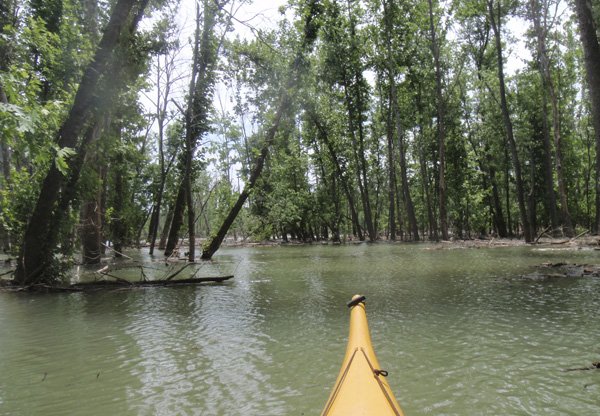The image captures a serene, greenish river or creek flowing gently through a town, as seen from the point of view of a person in a canoe. The yellow tip of the canoe, triangular and banana-colored, is visible at the bottom of the photo. Flanking the water are tall trees with dark trunks and vibrant green leaves, some of which lean towards the center, creating a lush canopy. The left side features prominently tall, thin black trunks emerging from the water, while the right side showcases a mixture of fallen branches and trees rooted on land. Above, the sky is a blend of blue and white, suggesting scattered clouds and a hidden sun. The overall scene embodies a tranquil outdoor adventure, evoking the sense of a peaceful, nature-filled expedition.